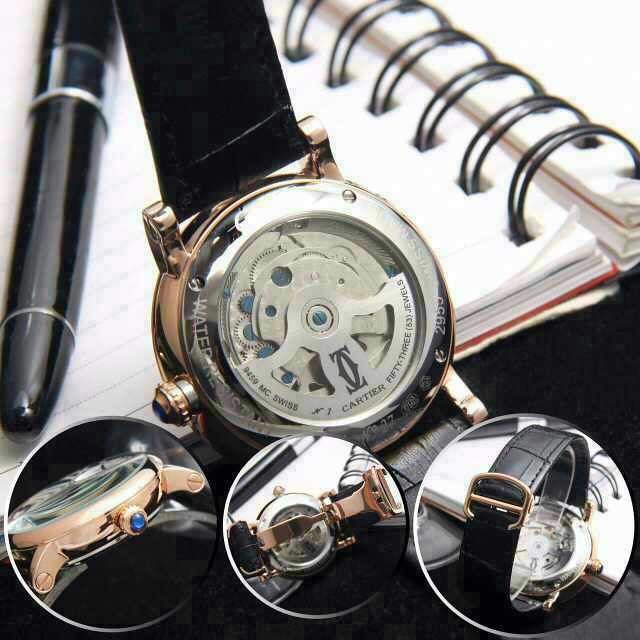A stunning timepiece takes center stage against the backdrop of an open spiral-bound notebook. The black spiral binding holds the two halves of the notebook together, while crisp white pages provide a clean canvas for an intriguing arrangement. A sophisticated black pen, exuding luxury and elegance, lies next to the showcased watch.

The watch itself commands attention with its golden bezel and intricate display of silver gears visible through the transparent back. The timepiece boasts a sleek black strap that is both stylish and modern. Enhancing its allure, three additional inset images offer distinct perspectives: 

1. A side view reveals the elegant golden edge and a striking blue jewel adorning the crown.
2. The face of the watch is displayed, showcasing an exquisite silver dial that complements the mechanical intricacies within.
3. The final inset depicts the watch face down, with the strap neatly buckled, highlighting a golden buckle that harmonizes perfectly with the watch's overall design.

This meticulous composition not only celebrates the watch's craftsmanship but also its aesthetic harmony with the surrounding elements.